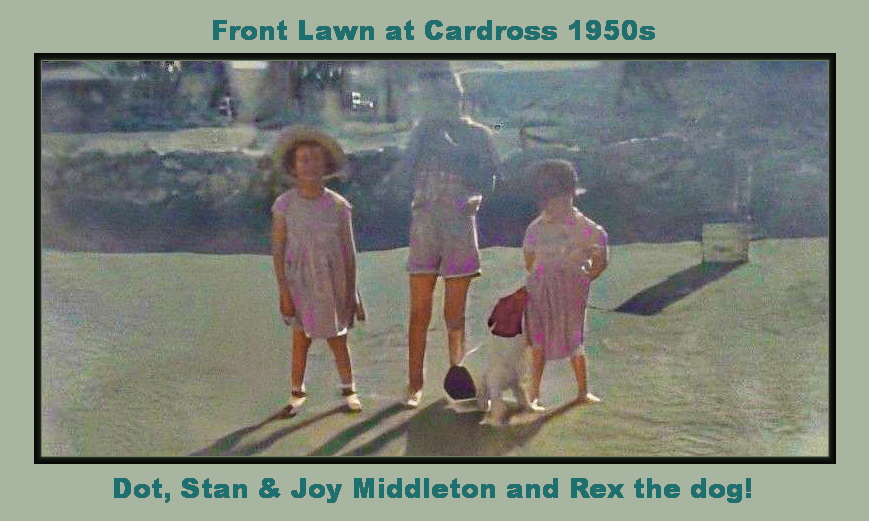This is an image of a photograph from the 1950s, bordered by a green frame with an inner thin black line. The text at the top of the border reads "Front Lawn at Cardross, 1950s," in a green sans serif font, while the text at the bottom reads "Dot, Stan, and Joy Middleton, and Rex the dog," also in green. The photograph shows three children and a dog standing outdoors, likely on a lawn. The child on the left is dressed in a pink dress with white shoes and a yellow straw hat. The middle child, who appears to be a girl but whose features are blurred due to the age and condition of the photo, is wearing a shirt with blue shorts and white shoes. The child on the right is also wearing a pink dress with white shoes. Positioned between the children in the middle and on the right is Rex, the dog. The aged photograph, which has a muted olive green background, shows the children standing on green grass under what seems to be bright sunlight, adding to the antique charm of the overall image.